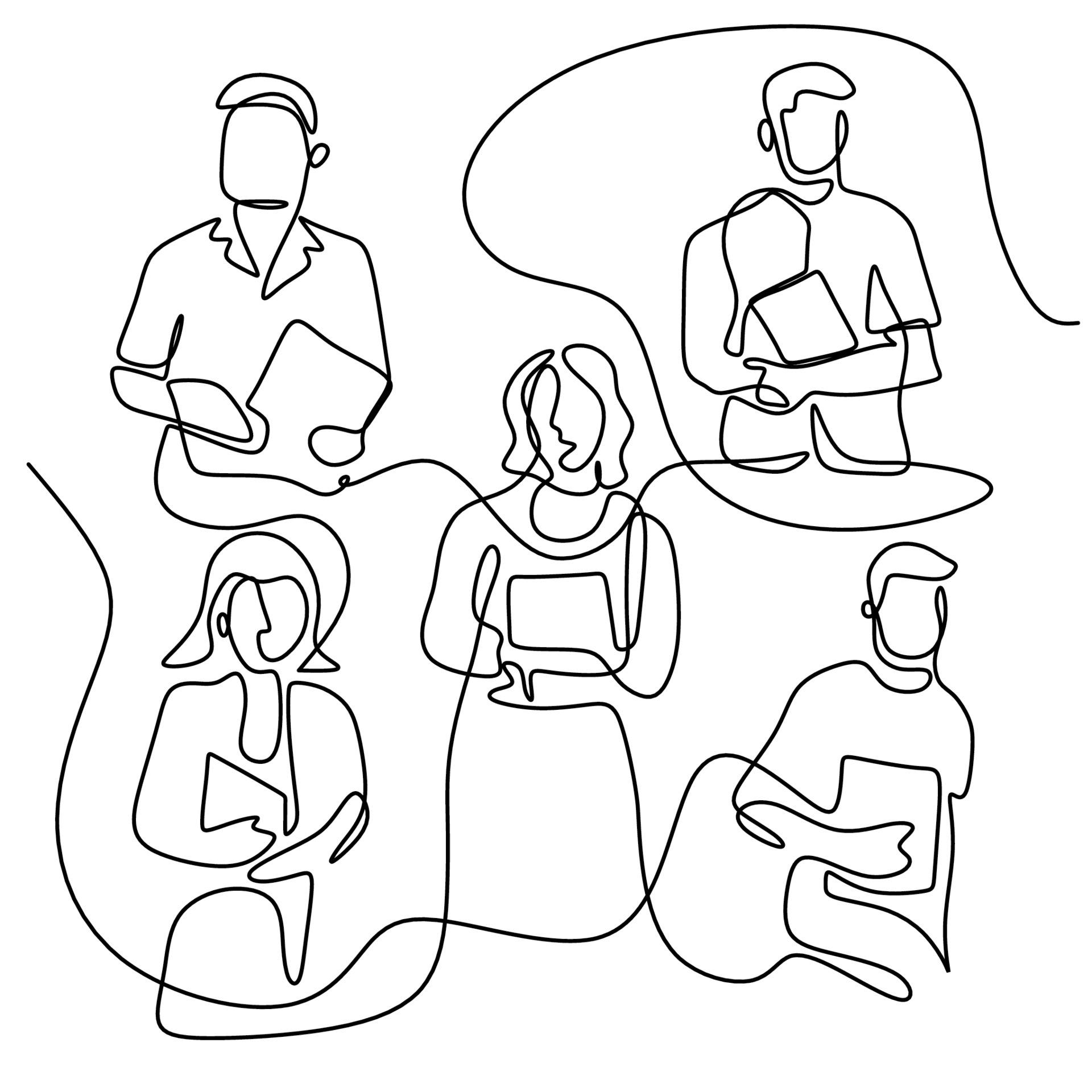This image is a black line drawing in a contemporary, popular squiggly and loopy artistic style. It features five faceless figures, three men and two women, all created from a continuous black line against a white background. At the center stands a woman with a slightly longer than bob haircut, dressed in a garment that loosely resembles a dress, and holding an indistinct object like a book, tablet, or folder. Surrounding her are four figures, each at the corner of the composition. In the top left corner, there's a man in a short-sleeved button-up shirt holding something akin to a folder. The man in the top right corner seems slimmer, wearing a t-shirt and clutching what could be a book or a small paddle. In the lower right corner appears a figure, possibly the same man from above but in motion, also holding a book in his right hand. Finally, the woman in the lower left corner is depicted mid-movement, holding an item. All figures are interlinked by the continuous black line and face the viewer, adding to the image's cohesive and dynamic aesthetic.